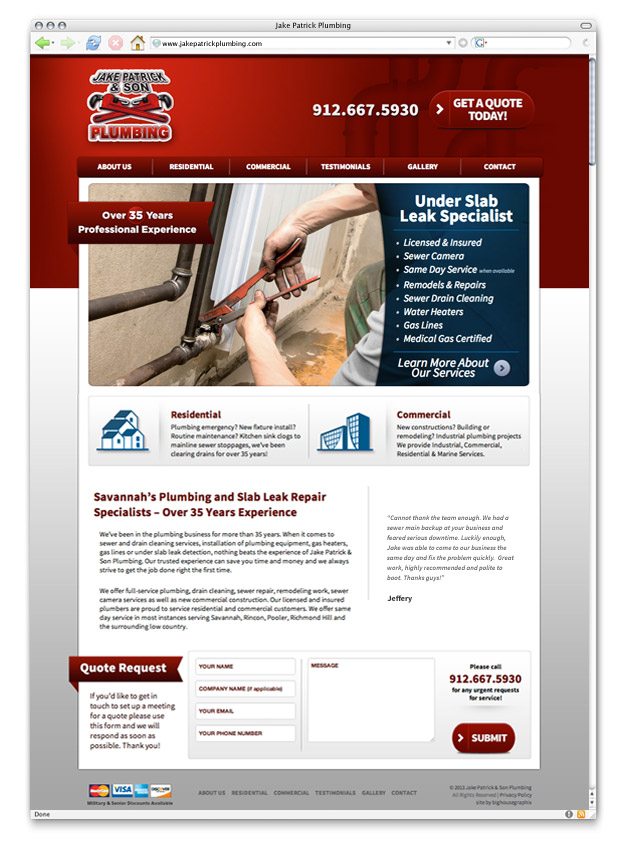The screenshot captures the homepage of Jake Patrick Plumbing's website, displayed within a web browser. The top section features a light gray header with a subtle gradient, transitioning from lighter at the top to darker at the bottom. On the far left of this header, there are three silvery orbs. Centrally positioned within the header, "Jake Patrick Plumbing" is written in black text. 

Beneath the header lies the URL bar, presented in white. A blue magnifying glass icon precedes the URL input field, where "www.jakepatrickplumbing.com" is typed. Adjacent to this, there's a gray downward-pointing triangle. Further to the right sits a search bar marked with a blue 'G' encased in a square.

To the left of the URL bar, there are several browser icons: a beige and brown house icon, a red circle with a white 'X' inside, two blue arrows forming a circle, a faded-out green right-pointing arrow, and a bright green left-pointing arrow.

The main website background is dual-toned, featuring a dark red gradient at the top and a white-to-light-gray gradient transitioning near the bottom. Stacked atop this background, the website content begins in the top left corner with a logo reading "Jake Patrick and Son Plumbing," flanked by two crossed red wrenches. The text "Jake Patrick and Son" appears in black, while "Plumbing" is in red.

To the right of the logo, the phone number "912.667.5930" is displayed in white. Next to the phone number is a dark red button featuring a white right-pointing arrow and the text "Get a Quote Today."

Below this section, there are navigation tabs in dark red buttons with white text, reading: About Us, Residential, Commercial, Testimonials, Gallery, and Contact. 

The main content area showcases an image of a plumber working with a wrench on a metal pipe. A dark red tag with white text overlays this image, stating "Over 35 Years of Professional Experience."